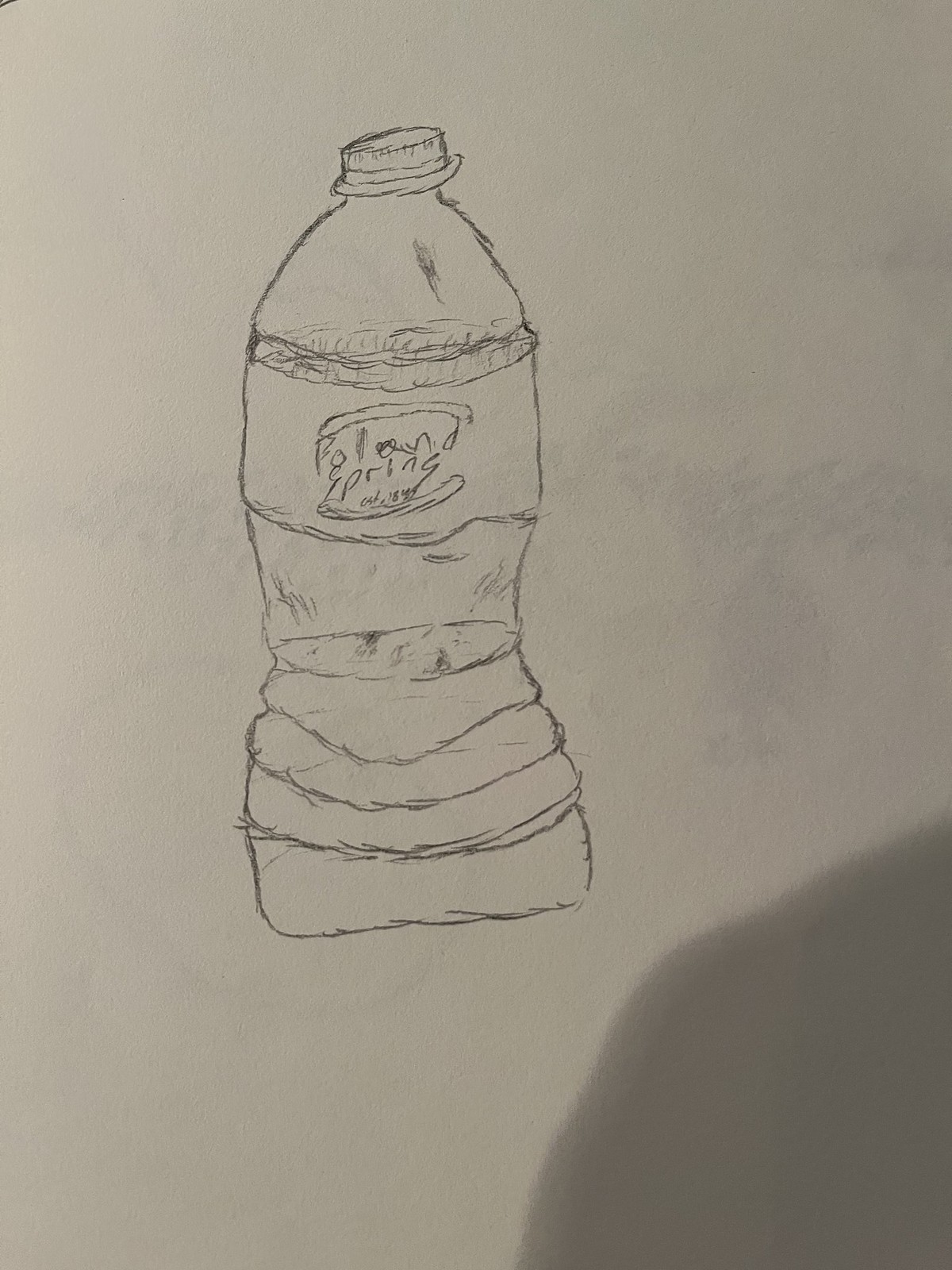This is a detailed portrait-style photograph of an illustration, capturing a sketch of a Poland Spring water bottle. The photo includes the cast shadow of the photographer in the lower right corner, indicating it was taken under direct light. The illustration clearly depicts the label text, although the top letters are somewhat indistinct, suggesting it's a branded bottled water. The artist has meticulously illustrated the bottle cap's ribbing, the bumpy texture at the base, and the remaining water inside, which is less than half full.